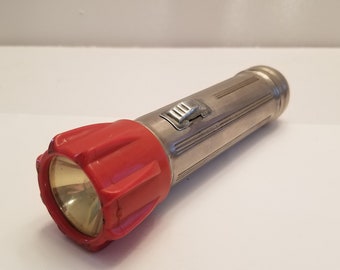This color photograph features a vintage-style flashlight set against an off-white background, lying on a white surface. The flashlight's handle and the button to activate it are made of silver metal, giving it a classic, sturdy appearance. The top section, which houses the light, is constructed of red plastic. The clear glass lens at the top reveals the silver metal interior and the tip of the clear light bulb, emphasizing its functional yet retro design. The flashlight appears to be of average, not particularly tall, size, adding to its utilitarian charm.